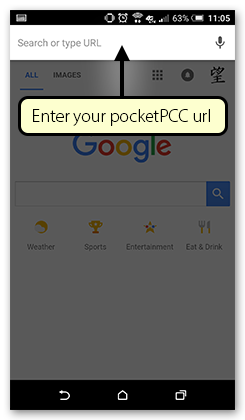The image appears to be a screenshot taken from a smartphone. At the top of the screen, there is a status bar displaying various icons. In the top-right corner, you can see the time, which is 11:05, followed by a battery icon showing a battery level of 63%. There are also icons indicating the strength of the signal and an alarm clock icon, along with a few others that are not easily identifiable.

Beneath the status bar is a search bar with a light yellow dialog box overlay reading "Enter your pocket PCC URL," with an arrow pointing up to the right. Directly to the right of the search bar is a microphone icon, suggesting the option for voice search.

Below this section, you will find the Google search interface. The page features the Google logo with Asian characters beneath it, indicating a user is signed in. There is the main search field where users can type their queries, accompanied by a blue magnifying glass icon for initiating the search.

Further down, there is a horizontal set of four emoji-like icons representing different categories: weather (globe icon), sports (trophy icon), entertainment (star icon), and eat & drink (fork and knife icon).

At the very bottom of the screen, there is a navigation bar with three main buttons in white against a black background. On the far left is a back button, in the middle is a home button, and on the right are double box icons for switching between apps or recent activity.